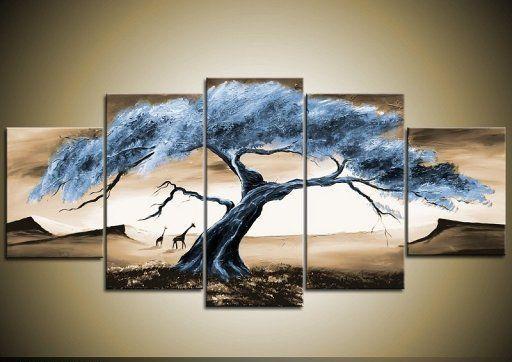The image depicts a detailed photograph of a painting divided into five individual sections of canvas, arranged from smallest on the outer edges to largest in the center, forming a pyramid-like structure. This multi-panel painting showcases a large willow or acacia tree that spreads across all five canvases. The tree appears to be dead, rendered in blue and blue-gray hues, set against a cream-colored background. The landscape features a dry, desert plain, likely resembling regions in Africa, with a couple of silhouettes of giraffes visible in the second section from the left. The overall color palette includes various shades of tan and blue, with a sky that transitions from dark clouds to a yellowed, pale hue. The painting is mounted on a wall colored in a gradient from black corners to a pale yellow center, adding depth and contrast to the scene. The tree leans slightly to the right, with additional details of sand dunes and subtle hills visible in the background.